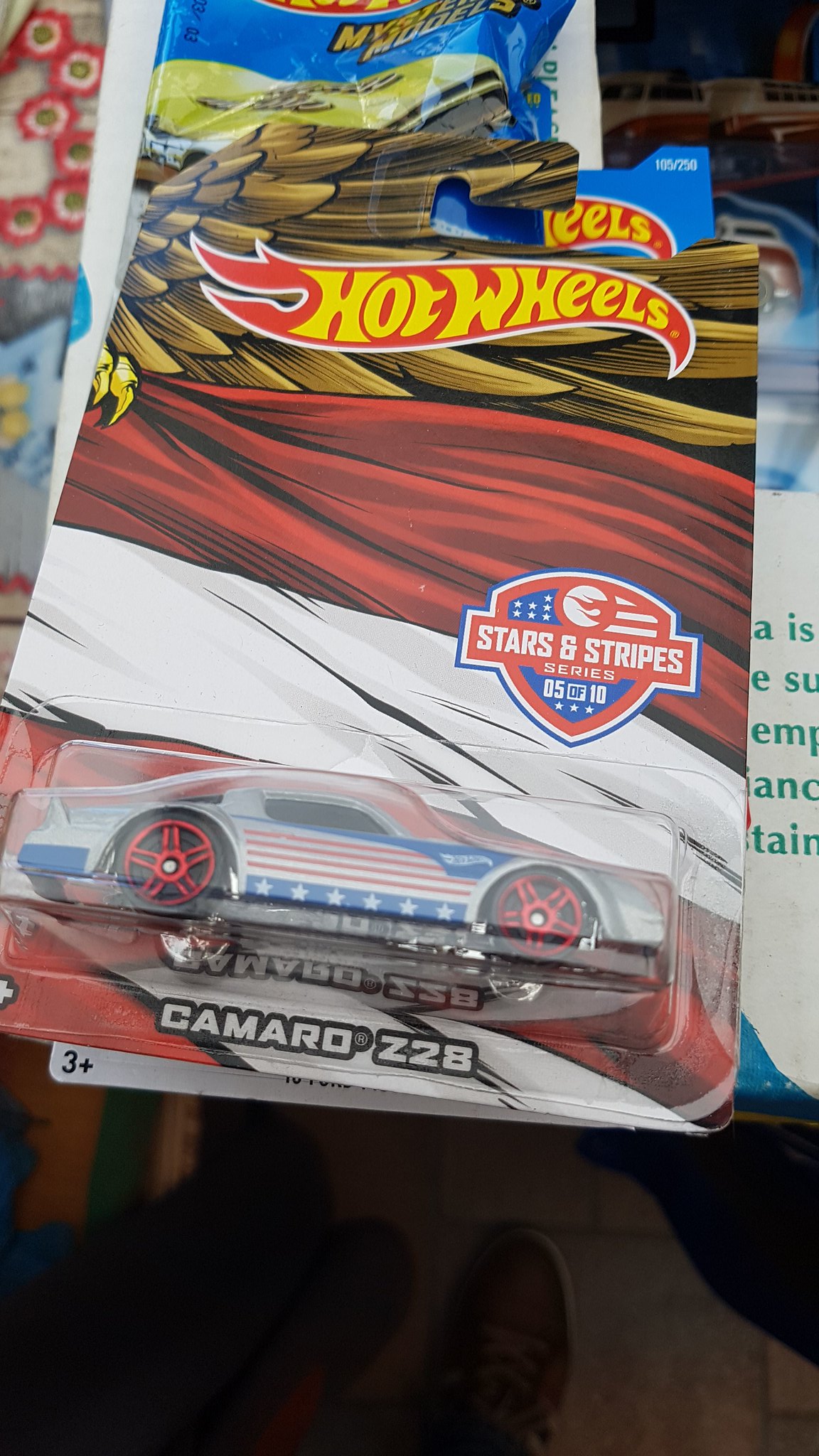The photograph captures a detailed scene of a Hot Wheels car in its original, unopened packaging, resting on a table. The setting appears dimly lit with the floor and a person's brown shoes visible in the background. The rectangular image, approximately six inches in height and three and a half inches in width, prominently features a Hot Wheels Stars and Stripes series car. The packaging's backdrop is a cardboard display with a natural hook for hanging.

At the top, a golden-winged eagle spreads across the packaging, clutching a flag with red and white horizontal stripes. The Hot Wheels logo, a prominent red banner with yellow print, overlays the eagle. Below, a red shield with a blue background and white stars enhances the patriotic theme. Clearly displayed within the plastic case is a white Camaro Z28 adorned with red, white, and blue stripes, along with snazzy red wheel spokes and star motifs.

The specific car is marked as part of the Stars and Stripes series, number five out of ten in the collection. In the background, another partially visible Hot Wheels package adds depth to the scene, and scattered red and white circles along with additional toy vehicles appear on the periphery. Text partially obstructed reads "A I S E S U E M A N T A I." The bottom of the image shows dark, indistinct objects, further contributing to the mysterious atmosphere.